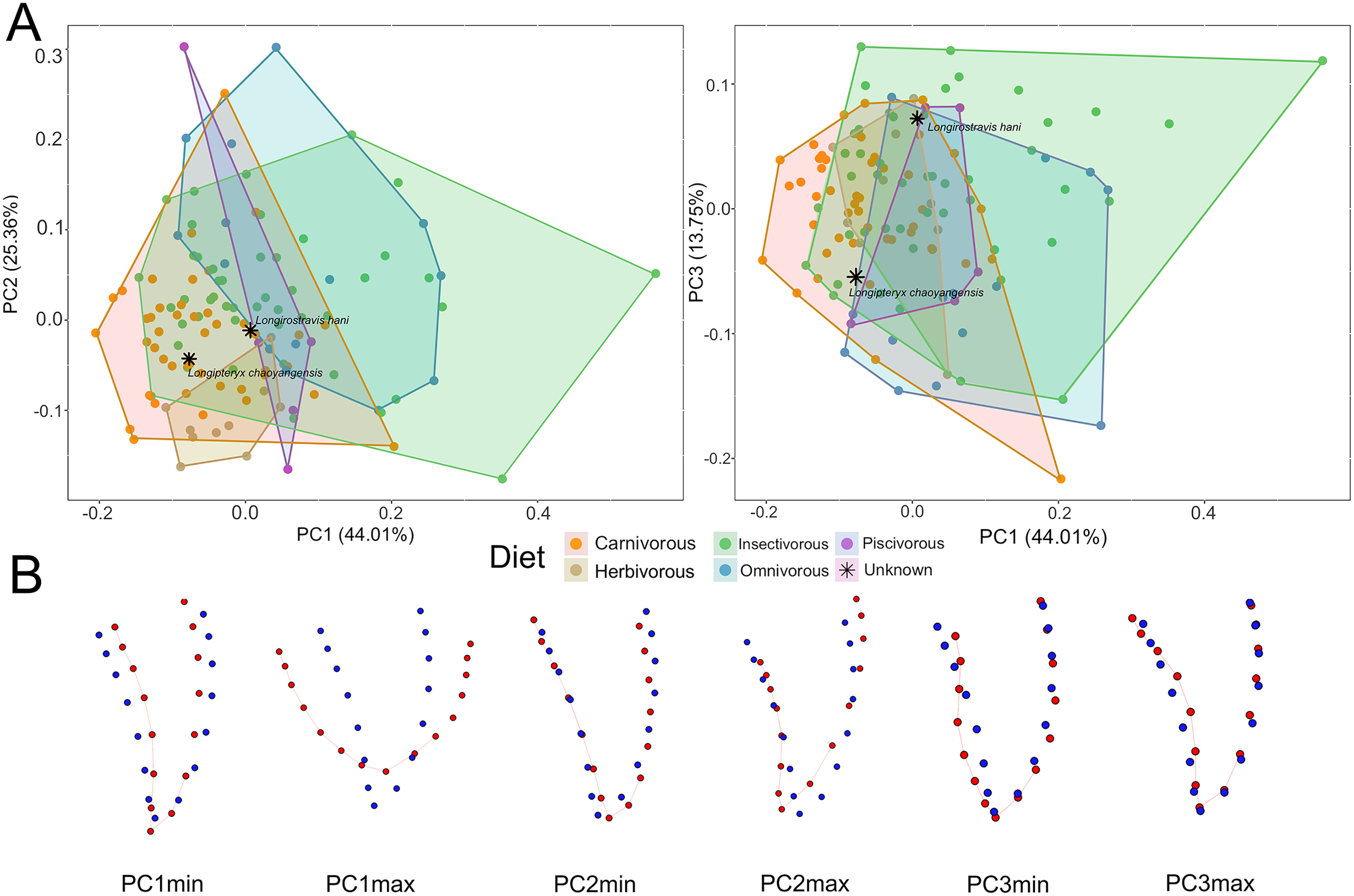The image features a detailed set of diagrams related to dietary classifications. At the top, labeled as "Exhibit A," there are two scatter point diagrams with colored shapes representing different dietary categories: yellow for carnivorous, light green for herbivorous, darker green for insectivorous, blue for omnivorous, purple for piscivorous, and an asterisk for unknown. The x-axis of the first diagram is labeled 'PC1 44.01%' and the y-axis as 'PC2 25.36%,' while the second diagram's y-axis is labeled 'PC3 13.72%'. 

Each graph showcases a variety of interlapping translucent colors, with dots scattered throughout to represent data points. The points are connected by lines forming differently colored shapes, which highlight the dietary categories.

Below these, labeled "Exhibit B," are six V-shaped graphs illustrating principal component analysis (PCA) results, shown with blue and red dots connected by lines. The x-axes and y-axes are labeled with PC1 min, PC1 max, PC2 min, PC2 max, PC3 min, and PC3 max. These graphs include numerical labels and show the distribution and variance within the respective principal components. 

Across all diagrams, the word "diet" is central, linking the data points to their respective dietary categories.